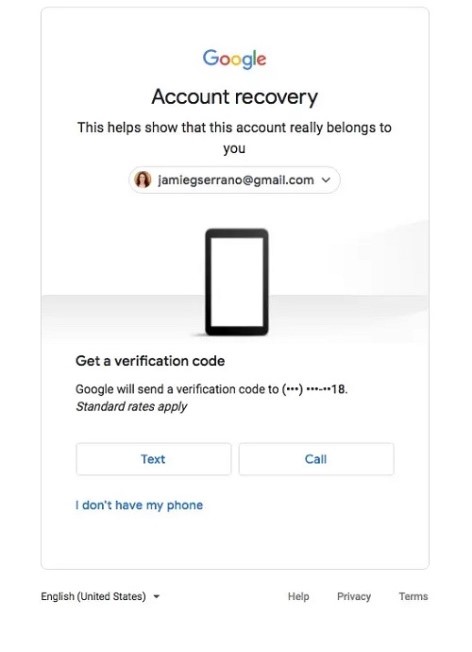This image is a screenshot of the Google Account Recovery page, likely displayed on a vertically-oriented tablet or mobile device. Dominating the screen at the top is the colorful Google logo, set against a stark white background. Directly below the logo, the bold, black text reads "Account recovery." Beneath this heading, a smaller caption in black states, "This helps show that this account really belongs to you," followed by an email address of the user undergoing the recovery process.

Centered on the page is an icon representing a mobile device or phone. Accompanying this icon is a directive, "Get a verification code," explaining that Google will send a verification code to the registered phone number. Most of this phone number is obscured with dots or stars for privacy. In addition, a disclaimer in italics cautions, "Standard rates will apply."

To receive the verification code, the user can choose between two blue buttons labeled "Text" or "Call." There is also a text option below these buttons reading, "I don't have my phone," providing an alternative recovery method.

At the bottom of the screen, users are presented with additional options, including switching the current language (English United States), seeking help, and viewing Google's privacy policy or terms of service.